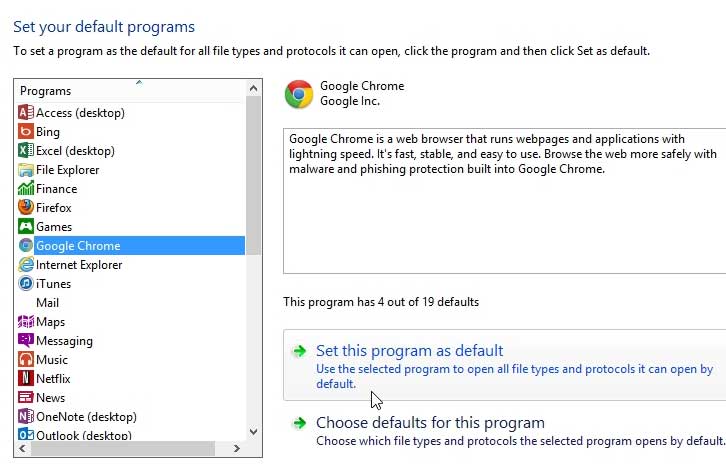A rectangular box occupies the central area of a predominantly white background, stretching horizontally from left to right. The box is neatly outlined in black with a vertical and horizontal scrollbar on the right edge and bottom edge, respectively. At the top-left corner of the box, there is a title in bold text: "Set your default programs." 

Beneath the title, a description guides the user: "To set a program as the default for all file types and protocols it can open, click the program and then click 'Set as default.'"

The main section of the box presents a list of program options arranged vertically on the left side, with the heading "Programs" above the list. The programs listed, from top to bottom, include Access, Desktop, Bing, Excel, Desktop, File Explorer, Finance, Firefox, Games, Google Chrome, Internet Explorer, iTunes, Mail, Maps, Messaging, Music, Netflix, News, OneNote on the Desktop, and Outlook on the Desktop. Notably, "Google Chrome" is highlighted in blue, with white lettering indicating its current selection. The scrollbar is positioned at the top, suggesting additional programs are available but not visible within the current view.

On the right side of the box, corresponding to the highlighted "Google Chrome" selection, there is a detailed description enclosed within a thin gray line. This section displays the Google Chrome icon and describes the program: "Google Chrome is a web browser that runs web pages and applications with lightning speed. It's fast, stable, and easy to use."